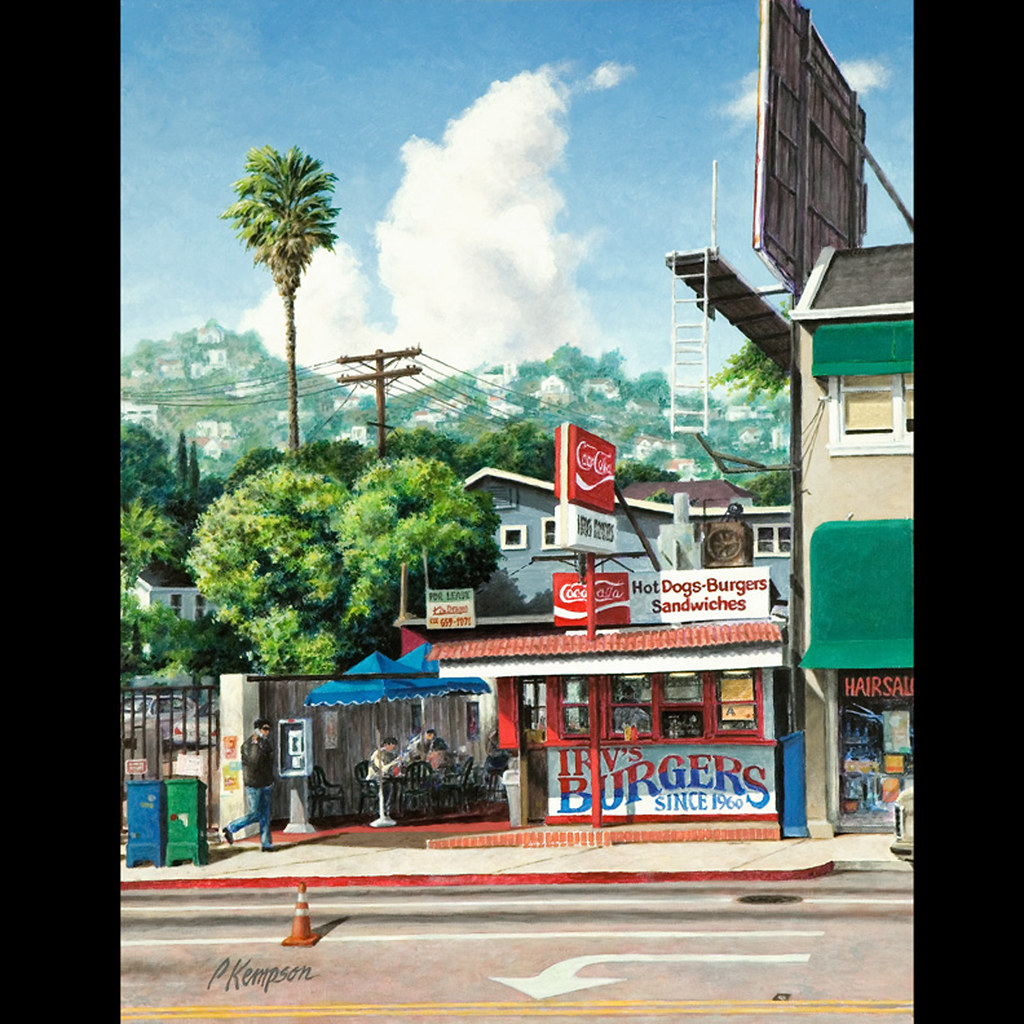The image is a detailed, full-color painting of a small, iconic burger restaurant named Irv's Burgers, established in 1960. The scene is set in a vibrant, neighborhood street view, framed by thick black bars on both the left and right sides. In the bottom left corner, the author's signature, P. Kempson, is visible, along with a small orange safety cone just above it.

The restaurant has a nostalgic red, white, and blue color scheme, accentuated by a red awning and several large Coca-Cola signs, including one prominent sign mounted on a red pole. The building displays the words, "Irv's Burgers, since 1960," and advertises "Hot Dogs, Burgers, and Sandwiches" in striking red text on a white background.

To the left of the restaurant, there's an outdoor seating area under blue canopies, where patrons can be seen enjoying their meals at tables. People are seated under umbrellas, adding to the cozy, communal atmosphere. In front of the building, a man wearing a black jacket is walking past a pay phone, engaged in a conversation on his cell phone.

The background of the image reveals a picturesque hillside with houses and green shrubbery, with a tall palm tree standing prominently behind the restaurant. The sky above is blue with scattered clouds, completing this charming neighborhood scene.